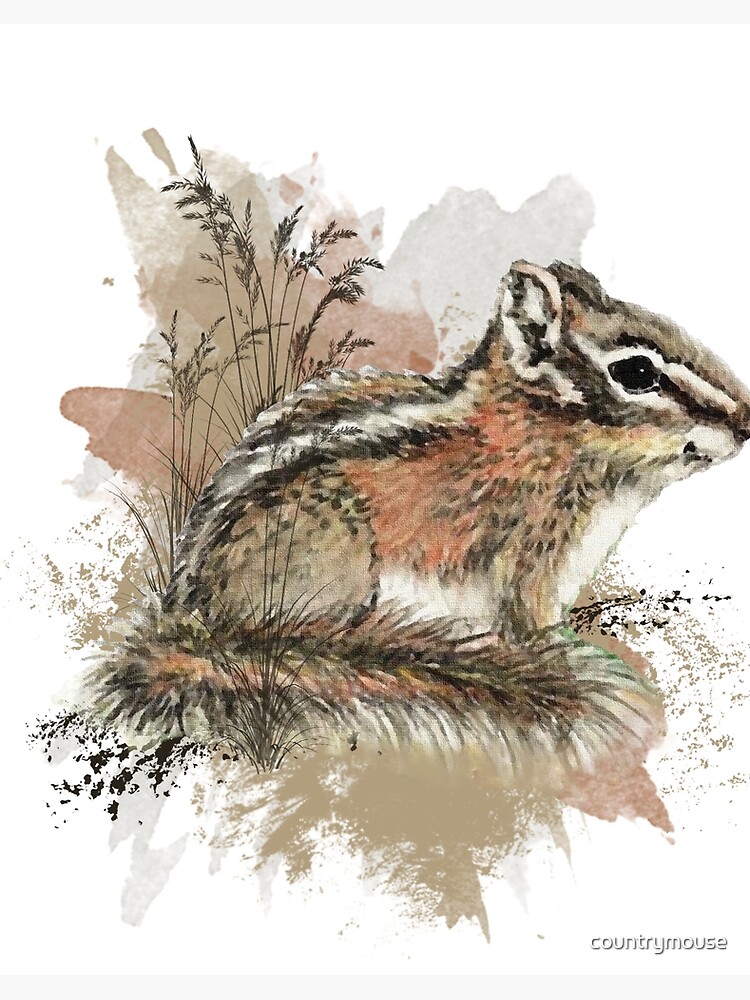This watercolor painting, reminiscent of illustrations found in a botany book, depicts a small rodent titled "Country Mouse" in the bottom right corner. The background is predominantly white with light gray, tan, and pink watercolor swatches scattered throughout, adding a splotchy texture. The animal, which appears to be either a chipmunk or a ground squirrel, faces right and is seated on a tuft of sparse grass and dried weeds. The rodent's coat features a complex palette, including shades of brown, pink, orange, yellow, and black. It has distinctive markings: black and white stripes down its back, white and brown ears, and a black eye encircled by white fur. The tail, characterized by wiry, wispy fur, is wrapped around its body, displaying hues of orange and black. Sparse foliage and blotches of color around the rodent contribute to the natural setting, encapsulating the essence of a delicate and detailed watercolor illustration.